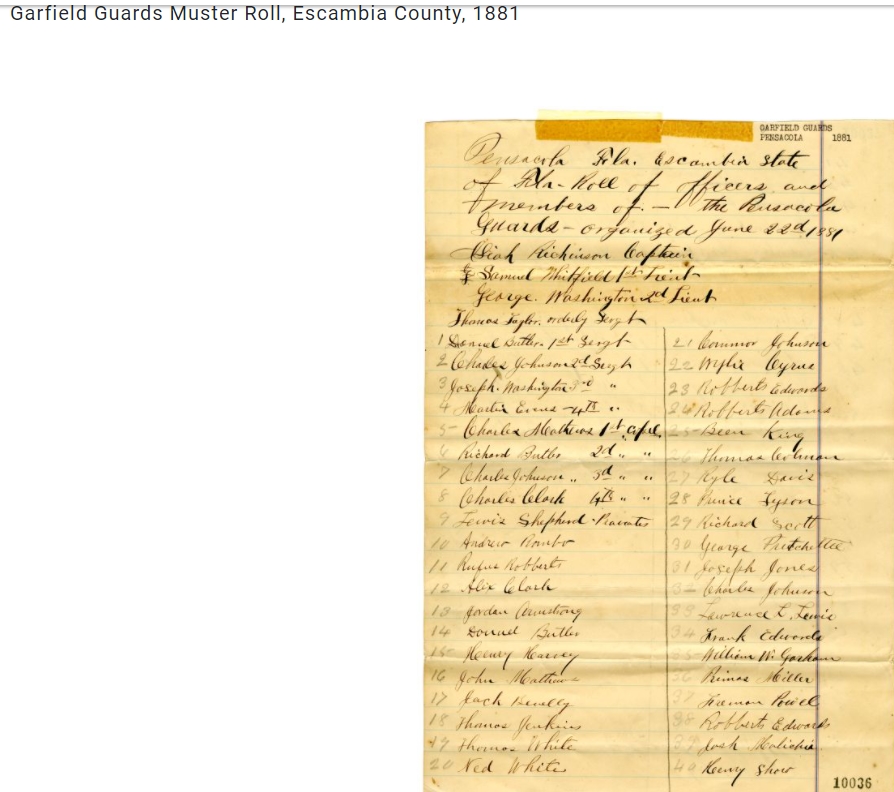The image depicts an old, yellowed piece of lined paper, possibly yellowed by age, resembling notebook or legal pad paper, with a prominent blue line running vertically down the right-hand side. The page features extensive cursive writing, primarily in black ink, and includes a list of names or signatures. The cursive is notably heavy and difficult to read, compounded by the poor quality of the image. The names are numerically listed, believed to range from 1 to 50 on one side and 21 to 60 on the other, although the exact numbering is not entirely clear.

At the top of the page, there is a handwritten title, "Garfield Guards at Escambia 1881," though this is also hard to decipher due to the heavy cursive. Additional text indicates that this is a muster roll of officers and members of the Pensacola Guards, organized in June 1881, in Escambia County, Florida. Three names of officers stand out in larger text: George Washington, Isaiah Richardson Caffrey, and Samuel Whitfield, although these too are somewhat difficult to make out.

A printed date in the top right corner indicates the year 1881. The bottom right corner features a numeral code, "10036." The overall condition of the document suggests it is quite old, with the lined paper potentially originally yellow or discolored from aging.